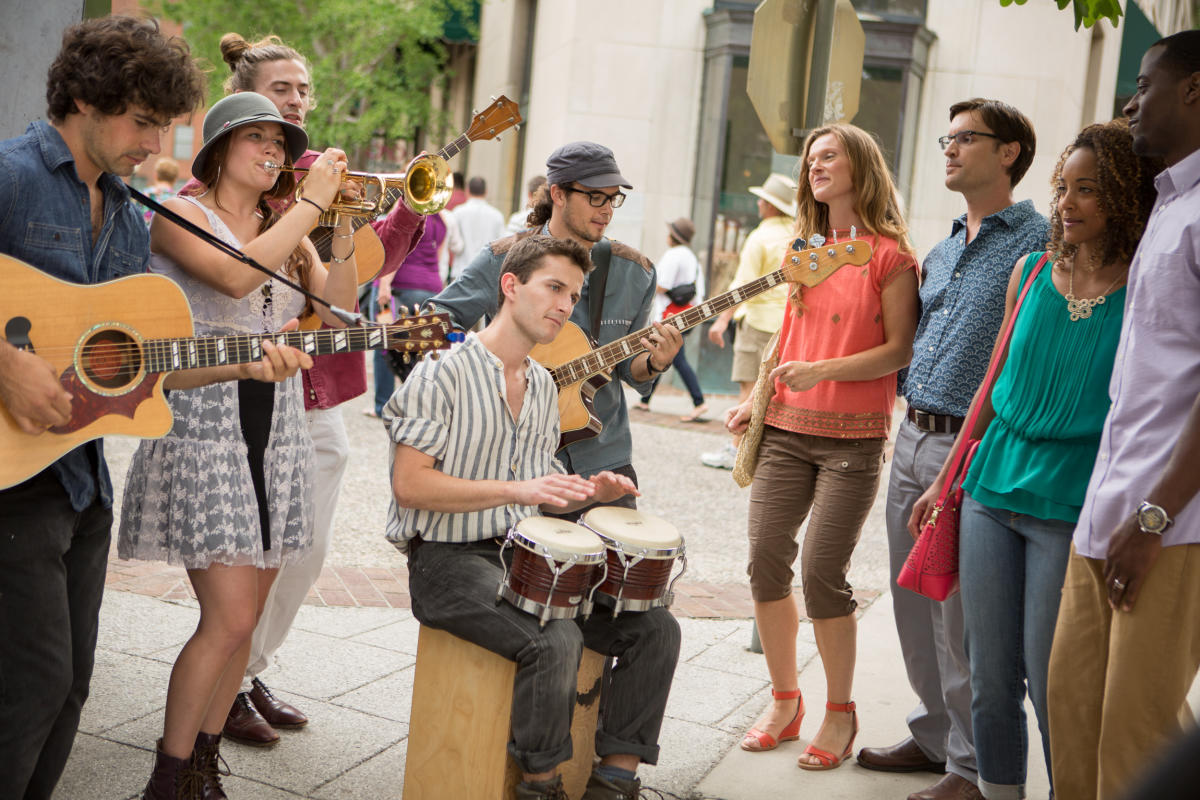In an outdoor scene, a lively group of street performers captivates a small crowd nestled on a city street in front of a beige building with a high, bronzy-colored doorway. Central to the image is a young man sitting on a yellow cube, playing bongo drums on his lap. He wears a white or beige and green-striped button-down shirt with sleeves rolled up, black jeans cuffed at the ankles, dark socks, and dark shoes partially cut off at the image's bottom edge.

Surrounding him are eight people, most involved in the musical performance while a few are simply observing. On the left, three guitar players contribute to the vibrant atmosphere: one man with long, curly brown hair, playing an acoustic guitar with a strap; a second man also with long hair tied up, clad in a taxicab hat and black-rimmed glasses, playing an electric-styled acoustic guitar; and a third male guitarist positioned right behind the bongos. A woman in a sheer white dress with a black patch and a navy blue bowler hat adds depth to the auditory scene with her trumpet. 

To the right of the central performer, four people—two women and two men—stand as part of the audience, attentively watching the performance. The harmonious interaction between the musicians and the onlookers brings a sense of community and enjoyment to the street, highlighting the universal appeal of music.